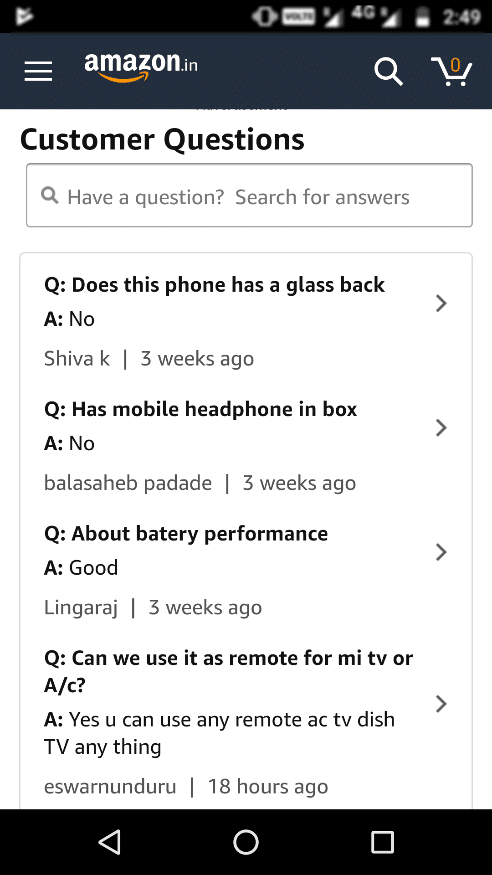This screenshot appears to be taken from a smartphone, displaying a section of the Amazon mobile application. The top portion of the screen shows the standard status bar, featuring icons from left to right: a triangular play button pointing to the right, an eye symbol, a small rectangular shape, a downward-pointing arrow, "4G" followed by a downward-pointing arrow, and a battery icon that is half full, accompanied by the time "2:49".

Beneath the status bar, there is a three-line menu icon, followed by the word "Amazon" in white with black print, and a shopping cart, indicating the app's main navigation elements.

The main content of the screen is centered around "Customer Questions" with a rectangular search bar below that reads "Have a question? Search for answers." This section contains a list of recently asked questions and their corresponding answers regarding a specific product:

1. **Question**: "Does this phone have a glass back?" 
   **Answer**: "No." 
   *Answered by: Shiva K, three weeks ago.*

2. **Question**: "Has mobile headphone in the box?" 
   **Answer**: "No." 
   *Answered by: Balasheeb Pidaid, three weeks ago.*

3. **Question**: "About battery performance?" 
   **Answer**: "Good." 
   *Answered by: Lingarj, three weeks ago.*

4. **Question**: "Can we use it as a remote for my TV or AC?" 
   **Answer**: "Yes. You can use any remote, AC, TV dish, TV, anything." 
   *Answered by: Nswarnundru, 18 hours ago.*

At the very bottom of the screen, there is a black rectangular box with three icons: a left-facing triangle, a circle, and a square, which are standard navigation buttons on many Android phones.